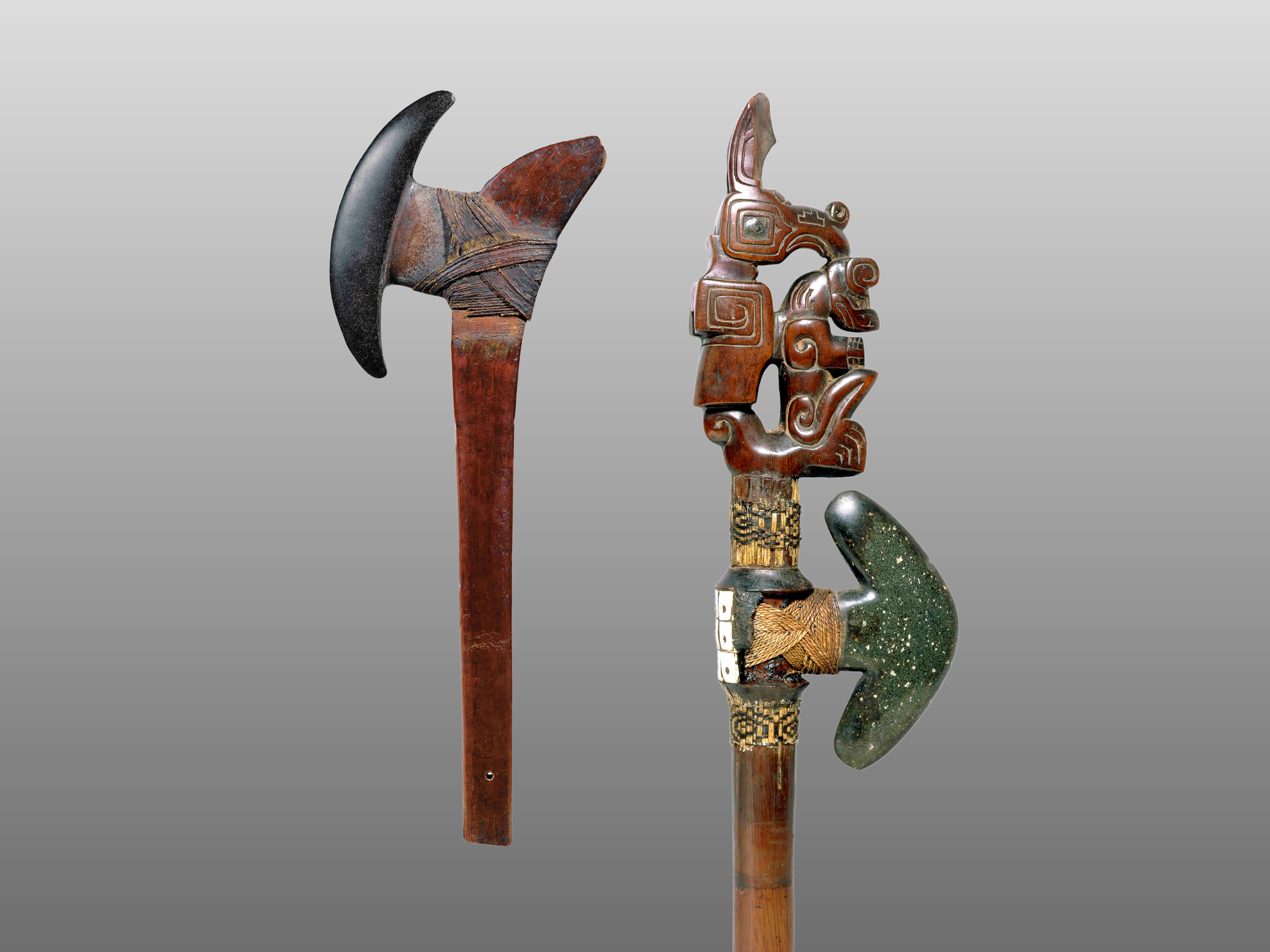The image depicts what appear to be old, possibly ceremonial tools or weapons, set against a bluish-gray background. To the left, there is an object resembling a tomahawk with a wooden handle and a black, crescent-shaped head that could be obsidian or a similarly dark stone. This head appears dull, potentially due to age, and is affixed to the handle with wrapping material that looks like twine or rope. To the right, another object might be a more ornate ceremonial axe or a club. This piece has an elaborate handle and features an intricate design at the top, depicting what seems to be a figure of an animal, possibly a rabbit or jackal, with another figure beside or on it. Below this ornate section is a green- and white-speckled stone, shaped somewhat like an arrowhead, though it also appears dull. The handles of both items are wooden and show significant wear, suggesting they are quite old.